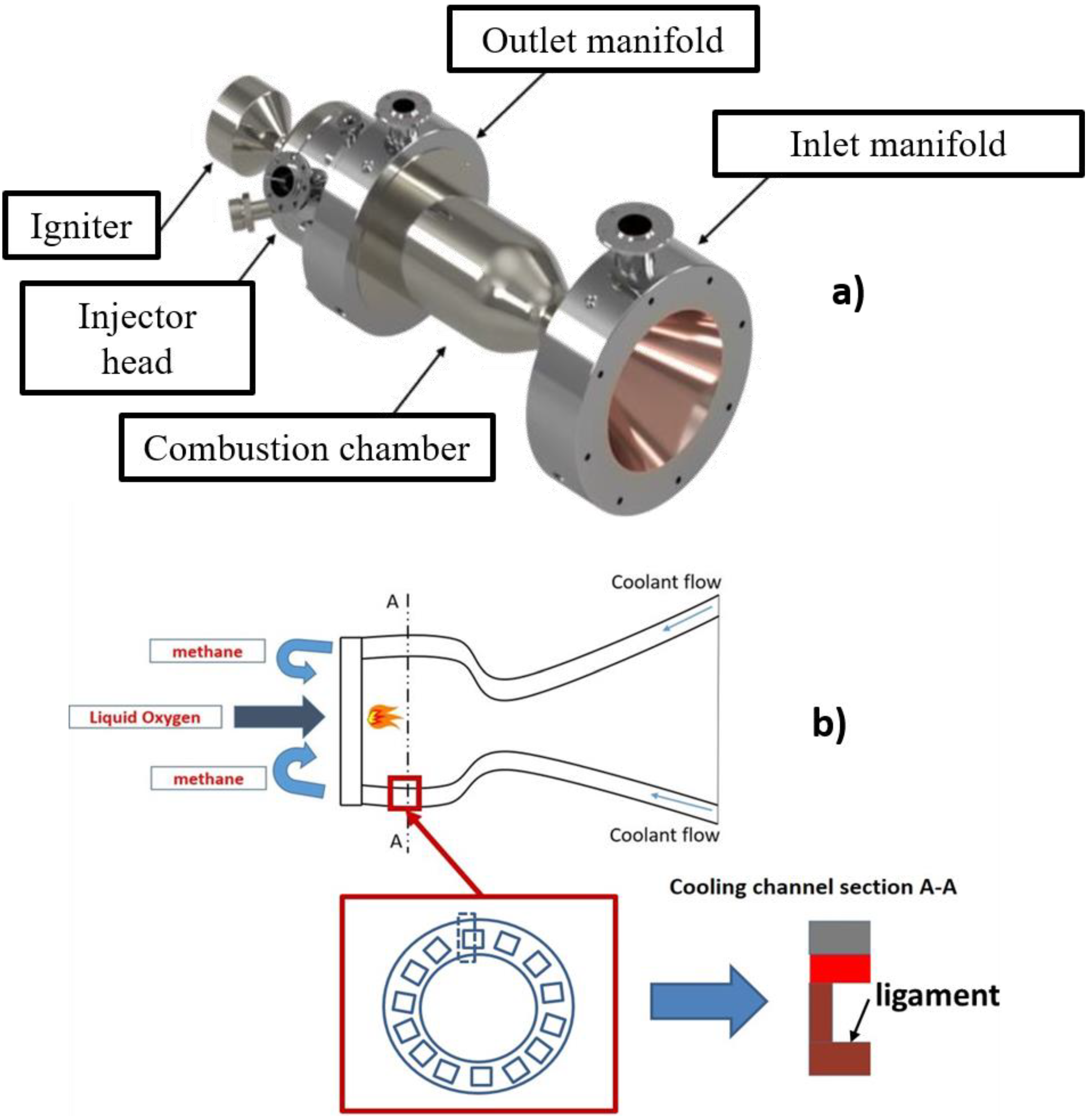This image depicts a detailed technical drawing of a cylindrical engine part, presented with a combination of color photograph and illustration, all set against a stark white background that creates a floating effect. The rectangular photograph is oriented such that its left and right sides are twice the length of the top and bottom edges. Positioned at an angle with the tip facing the top left and the head the bottom right, the engine part features multiple tubes, cylinders, and a prominent conical inlet on the bottom right.

The image is enriched with numerous informational labels in white rectangles bordered by black lines and containing black text. At the very top, the label reads "Outlet Manifold," directly beside it, "Inlet Manifold." As you move clockwise around the part, the labels identify "Combustion Chamber," "Injector Head," and "Igniter." 

Towards the bottom of the image, an additional diagram depicts the same engine part with further blowout labels and arrows pointing to specific sections. This diagram includes text such as "Methane," "Liquid Oxygen," and "Coolant Flow," rendered in red. There is also a detailed enlargement in a red square at the bottom, featuring another illustration highlighted by a blue arrow and a blue circle. Further down, letters "A" and "B" in parentheses are present, along with a color-separated rectangle in dark gray, red, and dark brown sections on the right.

Overall, the image combines photographic realism with illustrative elements to provide a comprehensive and labeled breakdown of the metal machine part’s various components and functions.